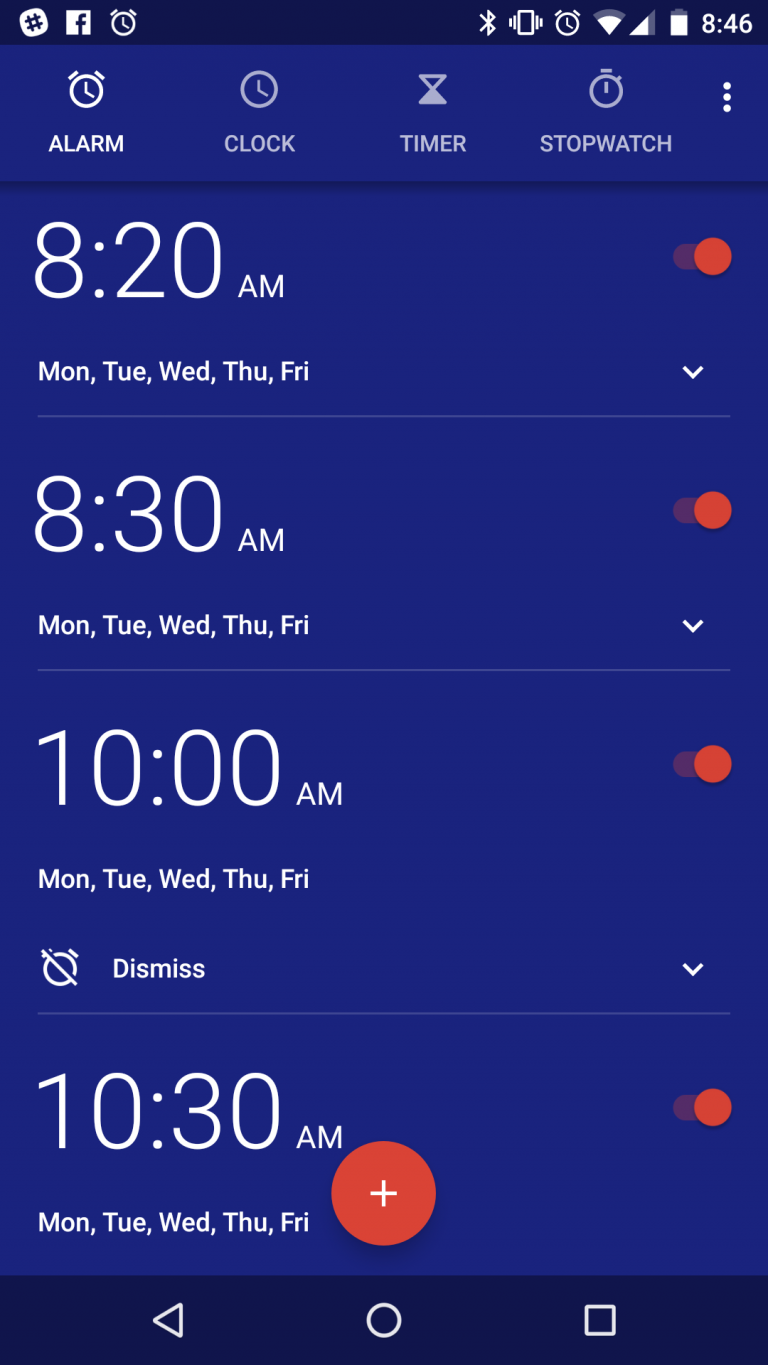The image is a screenshot from a cell phone displaying a web page. At the very top of the screen are several icons, including a rounded square with a hashtag symbol, the Facebook icon, and a clock icon. On the right side, additional symbols are visible, such as a clock, Wi-Fi signal, cellular bars, battery indicator, and the current time, 8:46.

In the main portion of the screenshot, the alarm function is selected. Below this, there are four alarms set for various times. The first alarm is set for 8:20 AM and is active from Monday to Friday. The second alarm is set for 8:30 AM, also active from Monday to Friday. The third alarm is set for 10:00 AM with the same weekday schedule, and it includes an icon of an alarm clock crossed out with the word "Dismiss" underneath the days of the week. The fourth alarm is set for 10:30 AM and is active from Monday to Friday. 

At the bottom of the list of alarms, there is a red circle with a plus sign, suggesting that additional alarms can be added or there are more alarms if scrolled down.

Finally, the screenshot shows the navigation bar of the phone at the bottom, which includes a triangle (back button), a circle (home button), and a square (recent apps button).